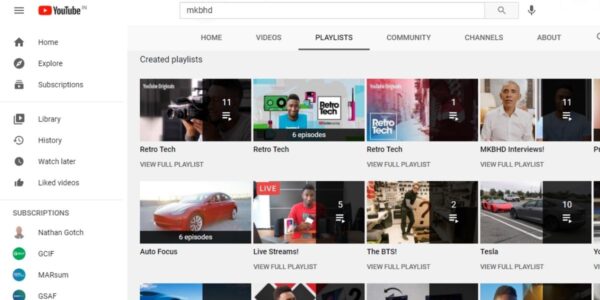This image is a screenshot of a YouTube page. On the left side, there is a sidebar that begins with the YouTube logo at the top. Directly beneath the logo are various navigation buttons, each accompanied by an icon to their left. The first section contains three buttons, followed by a horizontal divider line. Below this line are four more buttons, next to which "Subscriptions" is listed along with four channel links. The buttons listed in the sidebar include Home, Explore, Subscriptions, Library, History, Watch Later, and Liked Videos. Under the "Subscriptions" section, channels such as Nathan Gotch and C are visible, alongside three other channels.

The top right section of the page prominently features a search bar with "MKBHD" entered into it. The overall screen is predominantly white. Below the search bar, there is a set of six navigation tabs: Home, Videos, Playlists, Community, Channels, and About. The "Playlists" tab is currently underlined, indicating that it is selected. The main content area shows created playlists displayed in a grid format, consisting of three rows of video thumbnails.